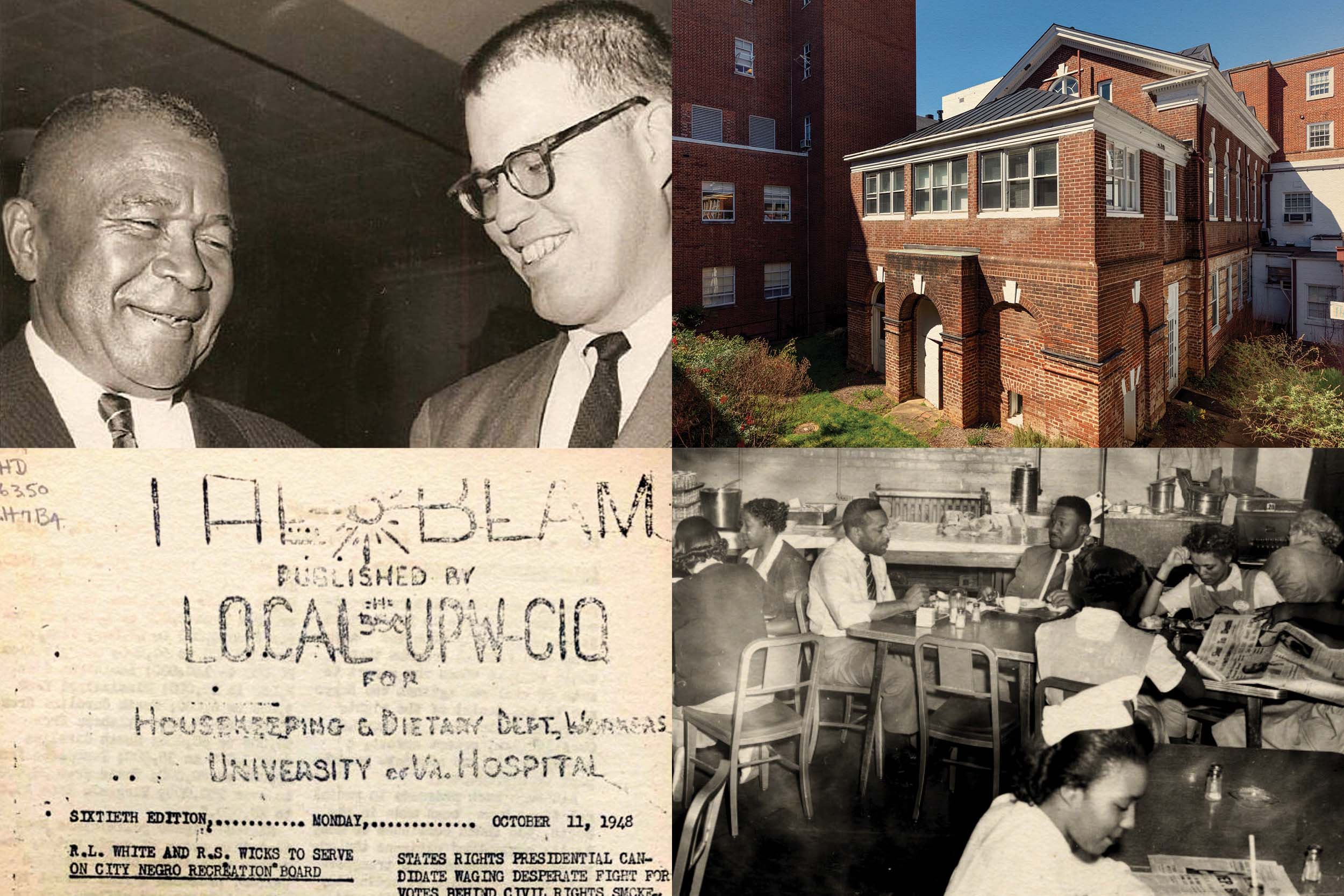This horizontal rectangular image is divided into four equal smaller rectangles, arranged in a grid with two on the top and two on the bottom. In the upper-left section, there's a photograph of two men in suits conversing; the younger white man on the right wears rimmed glasses, while the older black man on the left smiles beside him. The upper-right section features an image of an old red brick building that appears to be quite solid and is connected to other buildings. The bottom-left section consists of a faded and largely unreadable newspaper article, mentioning something about local housekeeping and dietary departments of workers possibly linked to the University of Virginia Hospital. Finally, the bottom-right section shows what appears to be a group of people, likely nurses, sitting and dining in what seems to be a hospital cafeteria or a restaurant.